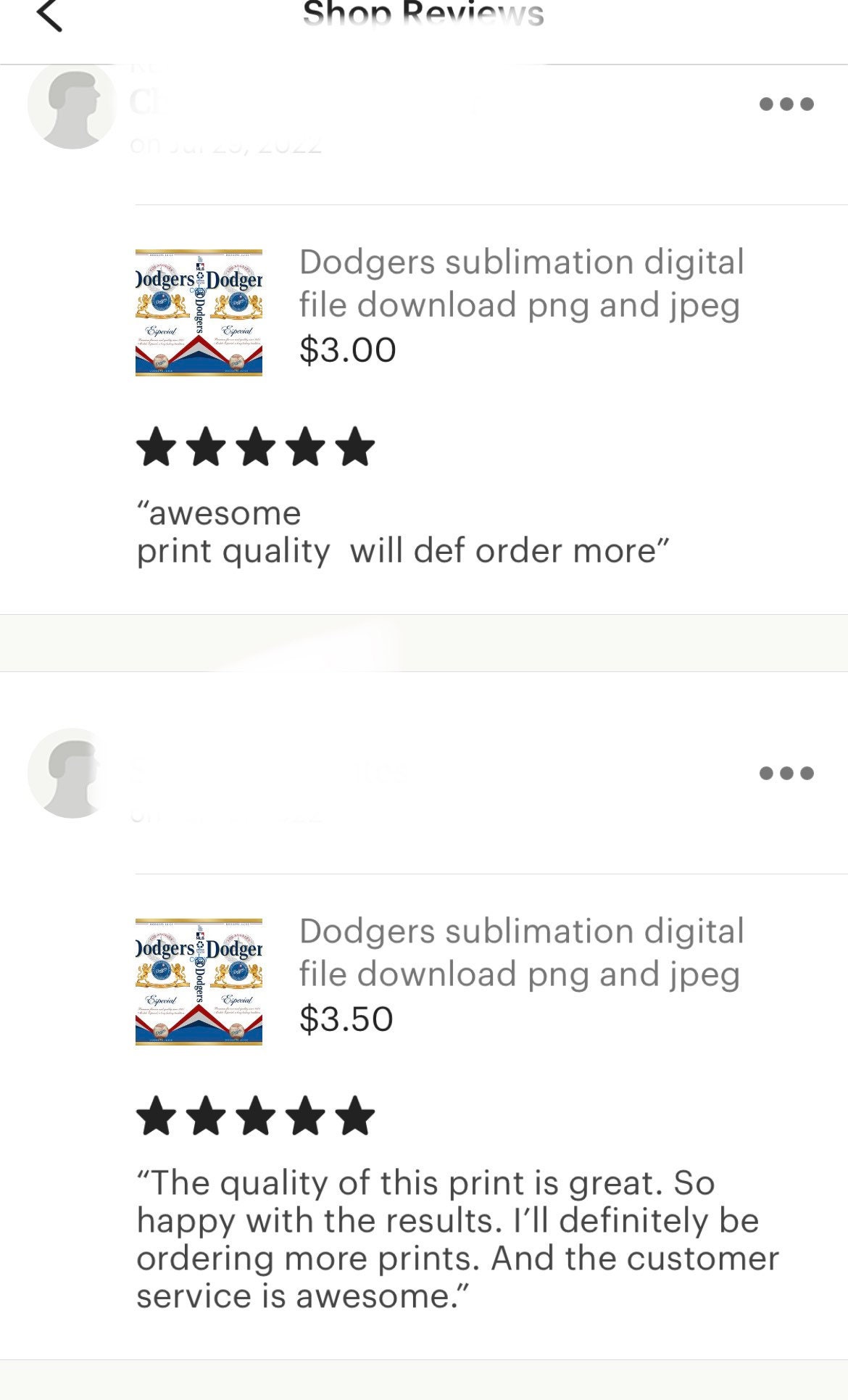This image showcases a review page most likely from an online marketplace or digital store. The header at the top reads "Shop Reviews." Below that, there is an empty circular icon, suggesting that the reviewer has not uploaded a personal photo. The username "Dodger" is displayed next to the icon, with a description of the reviewed item: "Dodger Sublimation Digital File Download, PNG and JPEG, $3." The review is rated five stars, with a comment reading, "Awesome print quality, will definitely order more!"

Underneath the first review, there is another anonymous review for the same item, but this time listed at $3.50. This second review also has a five-star rating and includes a detailed comment: "The quality of this print is great, so happy with the results. I'll definitely be ordering more prints, and the customer service is awesome."

Both reviews emphasize the high print quality and positive customer experience provided by the seller, Dodger.